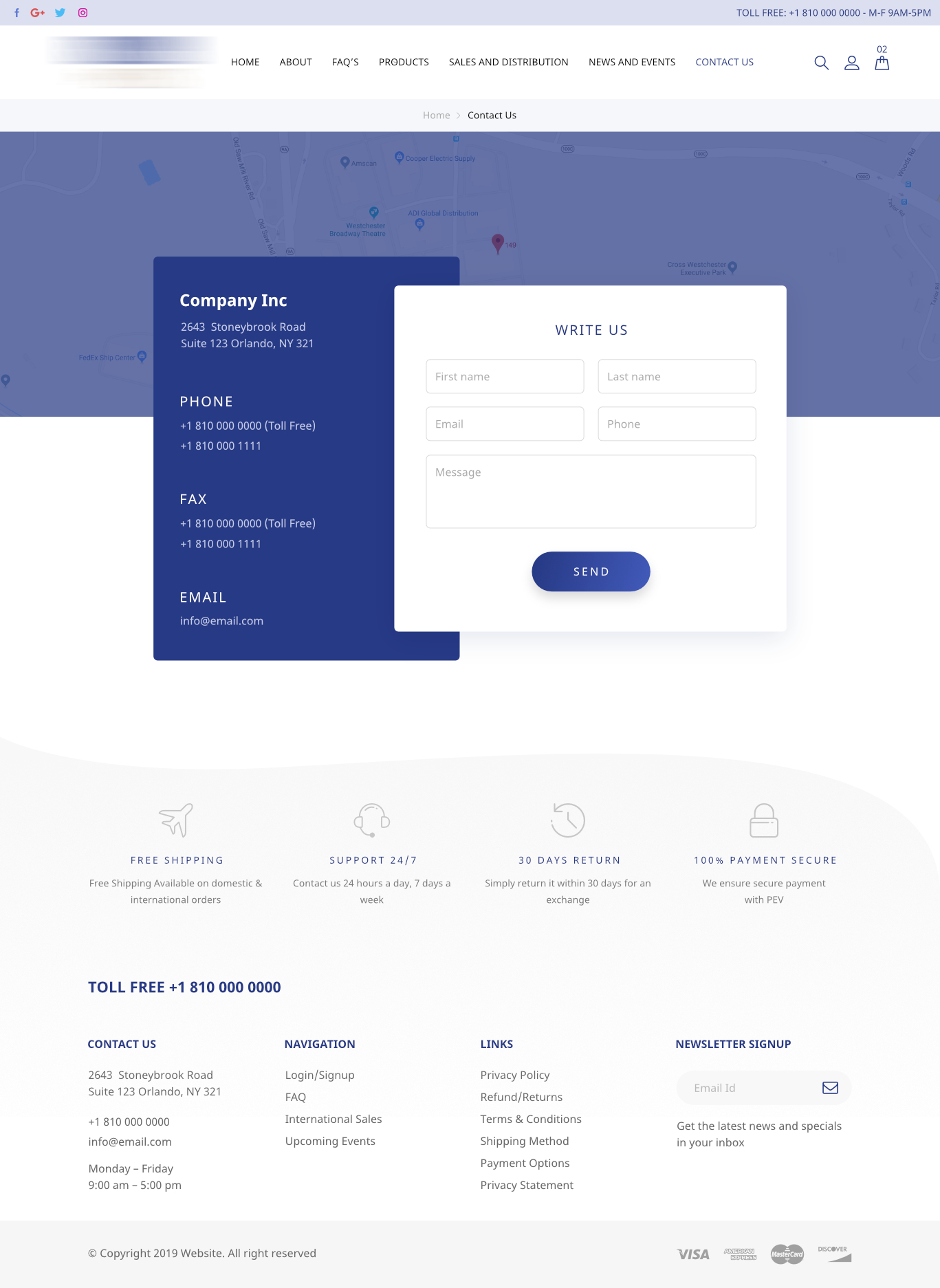This is a vertically-oriented screenshot from a user's computer screen or smart device, lacking a real-world background and using primarily white space. At the top of the image, a long, light purple-blue rectangle spans horizontally, containing social media icons on the upper left for Facebook, Google+, Twitter, and Instagram. Opposite these icons, on the upper right, are a toll-free number and the operation hours of the business.

Below this header, there is a squiggly, purple-white graphic element beneath the Instagram and Twitter icons. Centrally located in black text are navigation links for Home, About, Frequently Asked Questions, Products, Sales and Distribution, News and Events, and Contact Us. Adjacent to these links are icons for a search function, user account, shopping cart, and a shopping bag.

Further down, a pale purple bar repeats the Home and Contact Us links. Underneath, a map-like background gives way to a darker blue box detailing the company's contact information, including phone, fax, and email. Below this, there's a section titled "Write Us," featuring fields for the user's name and message, along with a send button.

At the bottom of the page, a gray box provides additional information, such as offers for free shipping, support, a 30-day return policy, and 100% payment security. It also reiterates the toll-free number and lists sections for navigation links, newsletter signup, and payment method details.